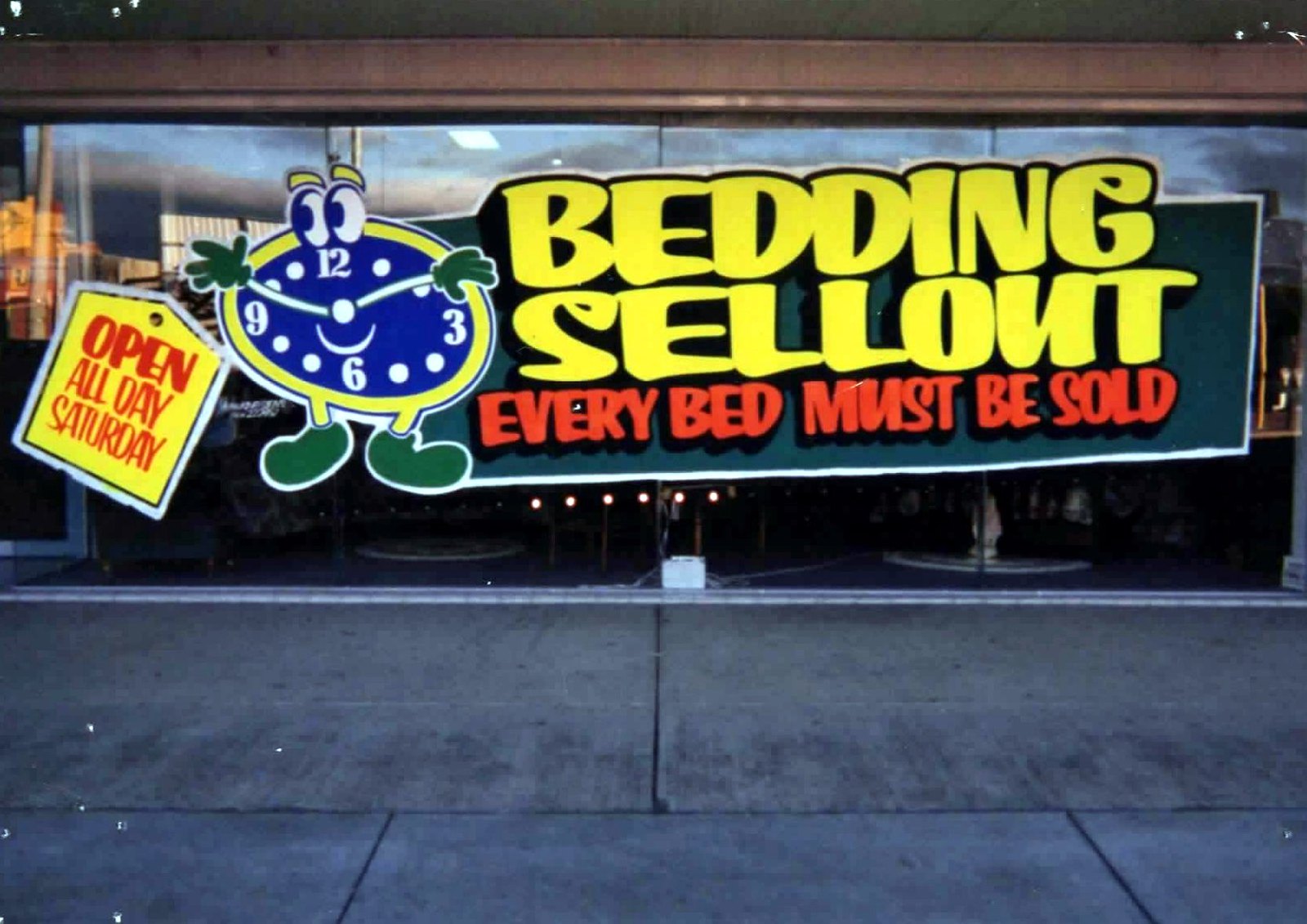The image shows a dimly lit exterior of a storefront with a wide, multi-pane glass window held in place by thin vertical frames. Painted on these glass doors, starting from the left, is an orange price tag with red letters stating "Open All Day Saturday." Adjacent to the tag is a large, animated blue clock with white numbers, yellow borders, and eyes with yellow eyebrows on top. The clock has anthropomorphic features, including green hands and feet. To the right of the clock, in bold yellow capital letters, is the text "Bedding Sellout," followed by "Every Bed Must Be Sold" in red capital letters. The scene includes a dark gray cement sidewalk in the foreground, with visible lines marking where people walk. Reflections of several buildings can be seen in the upper left of the window.